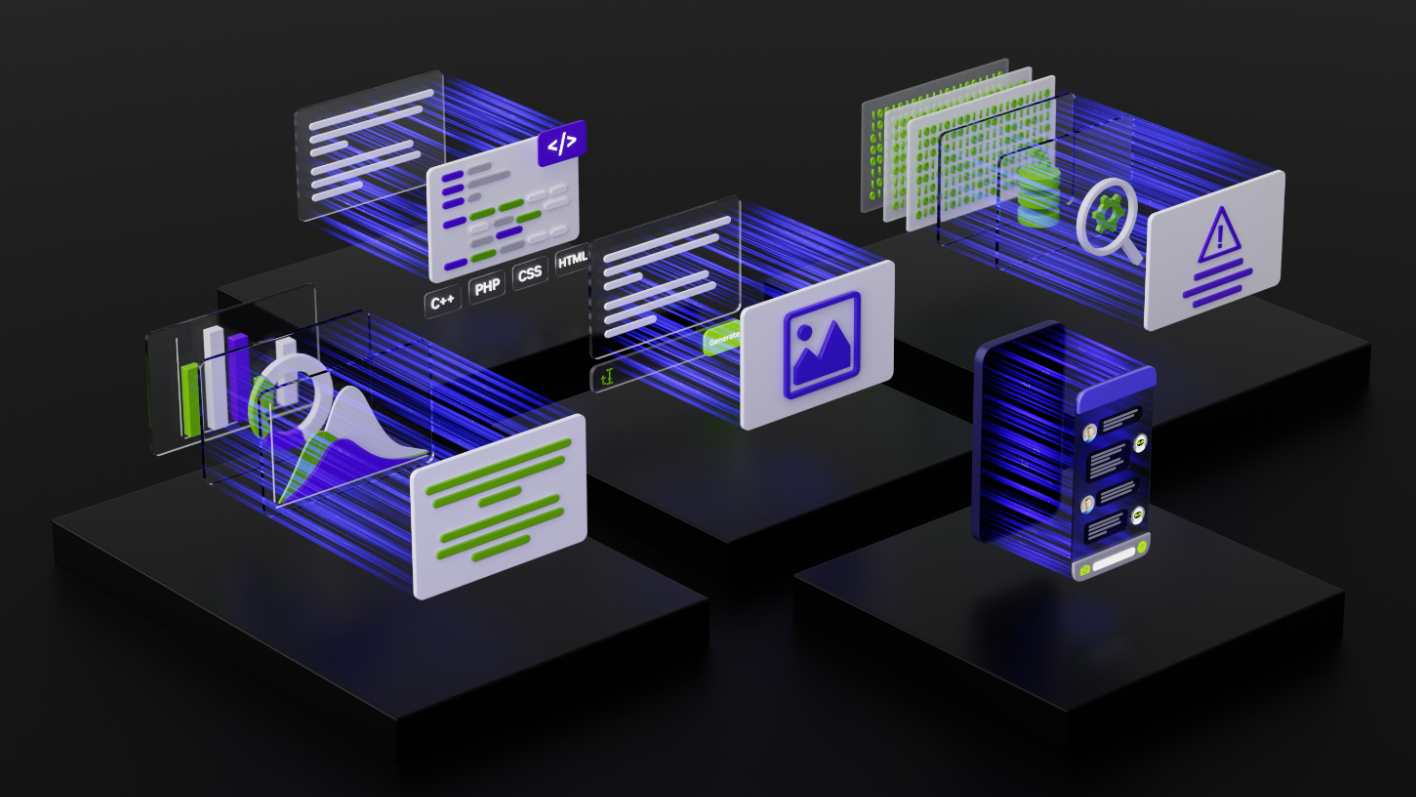This image is a detailed 3D digital illustration of various computer servers, arranged in a plus-sign formation on separate black platforms against a solid black background. Each server platform is adorned with distinct clipart icons to indicate its function: one features a cogwheel emblem for coding, another a database symbol for data storage, a third displays a landscape icon for photos, a fourth has a caution triangle for errors, and the fifth, positioned in the bottom right, shows a phone screen symbolizing messaging. Each server is interconnected by holographic, blue lines that traverse across the platforms, giving the impression of data flow and connectivity within a high-tech environment. The blue lines also form hollow cubes and intricate patterns behind each server, enhancing the futuristic and sophisticated aesthetic of the diagram.